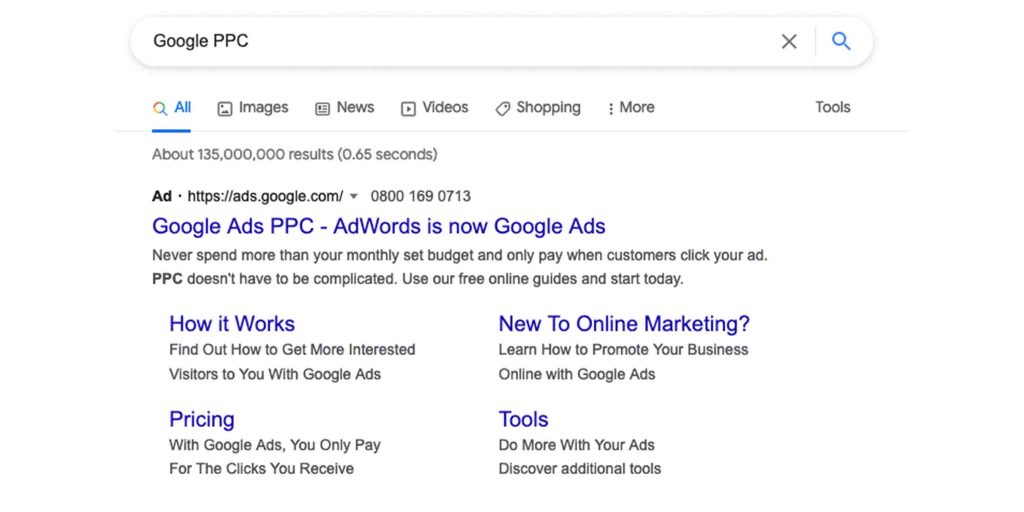The image is a screenshot of a Google search results page with a focus on Google PPC (Pay-Per-Click) advertising. At the very top, the page displays the text "Google PPC," followed by a search emblem. Directly beneath, there is a navigation menu with the options "All" (highlighted in red), "Images," "News," "Video," "Shopping," and "More."

Below the navigation menu, the search results indicate approximately "135 million results (0.65 seconds)." The primary result is an advertisement with an HTTPS address link to "ads.google.com." The blue-colored headline reads, "Google Ads PPC ad word is now Google Ads," followed by a black text description: "Never spend more than your monthly set budget. Only pay when customers click your ad. PPC doesn't have to be complicated. Use our free online guideline to start today."

Further down, there is a section with multiple bolded blue headings. The first heading, "How it works," is followed by the text, "Find out how to get more interested visitors to your Google Ads." The next heading, "Pricing," states, "With Google Ads you only pay for the clicks you receive." The final heading, "Tools," reads, "Do more with ads, discover additional tools." There is also a section titled "New to online marketing" which says, "Learn how to promote your business online with Google Ads," all in black text.

The entire background of the page is completely white, providing a clean and simple layout.